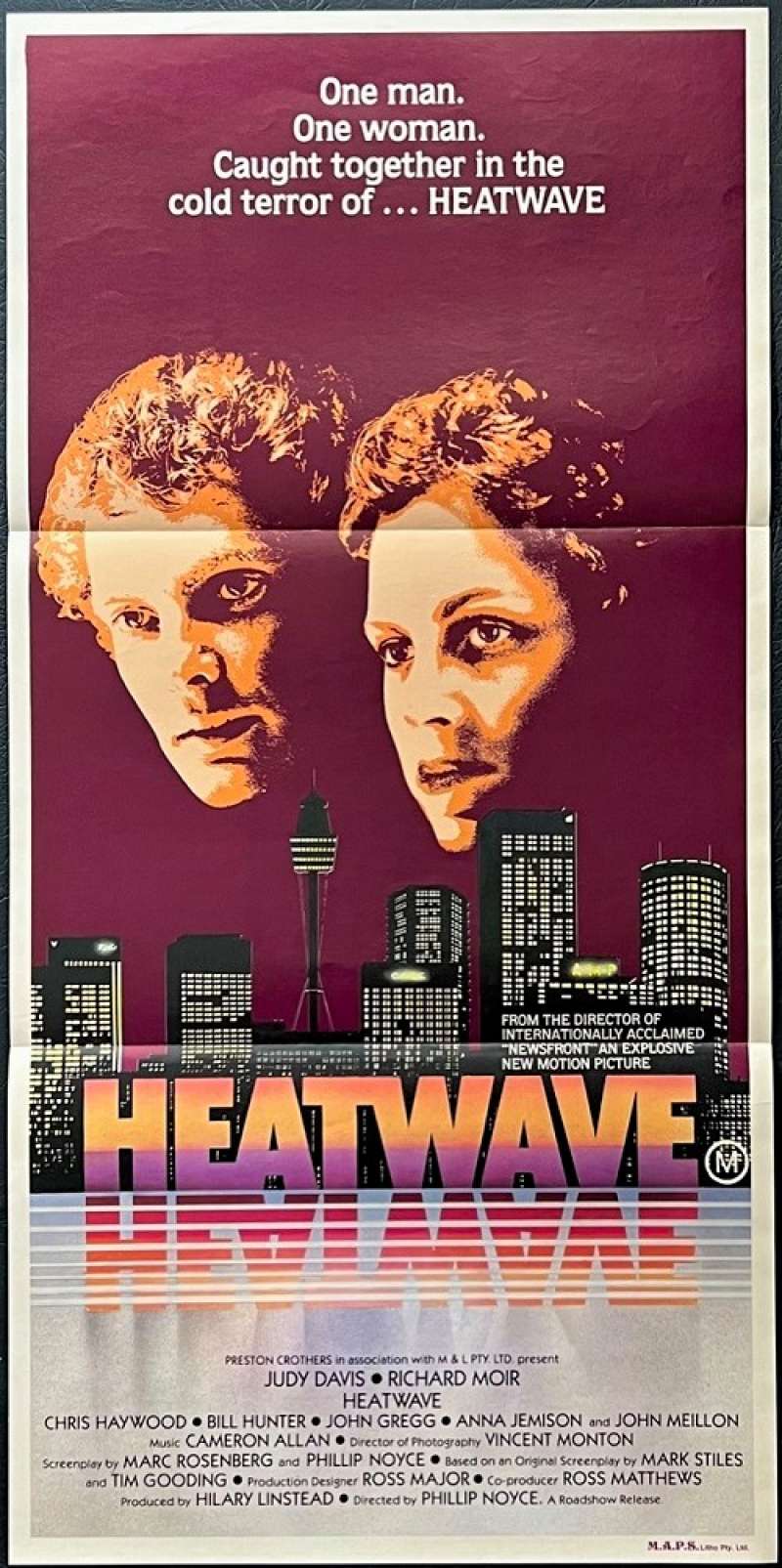The movie poster for "HEATWAVE" is a tall, narrow design, measuring approximately 11 inches wide by 25 1/2 inches long. Dominated by a rich purple background at the top, it draws immediate attention to the dramatic theme. Below this, the central section features a monochromatic black-and-white cityscape, enhancing the intensity of the visual narrative.

Above the cityscape, the serious expressions of the two leading actors, Judy Davis and Richard Moir, are prominently displayed. Their faces, shadowed and closely positioned, create a poignant centerpiece. Both actors have lighter curly hair and are gazing intently towards the left side of the poster, adding to the intriguing atmosphere.

A striking tagline in white font reads, "One man, one woman caught together in the cold terror of... HEATWAVE," setting an ominous tone for the film. The title "HEATWAVE" itself is boldly displayed in the same font, featuring a gradient of purple, orange, and melon colors, adding a vivid touch to the otherwise stark poster. 

Additionally, the title is reflected in a stylized water effect below the cityscape, merging seamlessly with the overall design. At the very bottom, the poster lists the names of the main cast and crew, including Judy Davis, Richard Moir, Chris Haywood, Bill Hunter, John Gregg, Anna Jemison, and John Mellon, among others. This detailed layout not only highlights the film's title and tagline but also provides essential credits for the contributors.